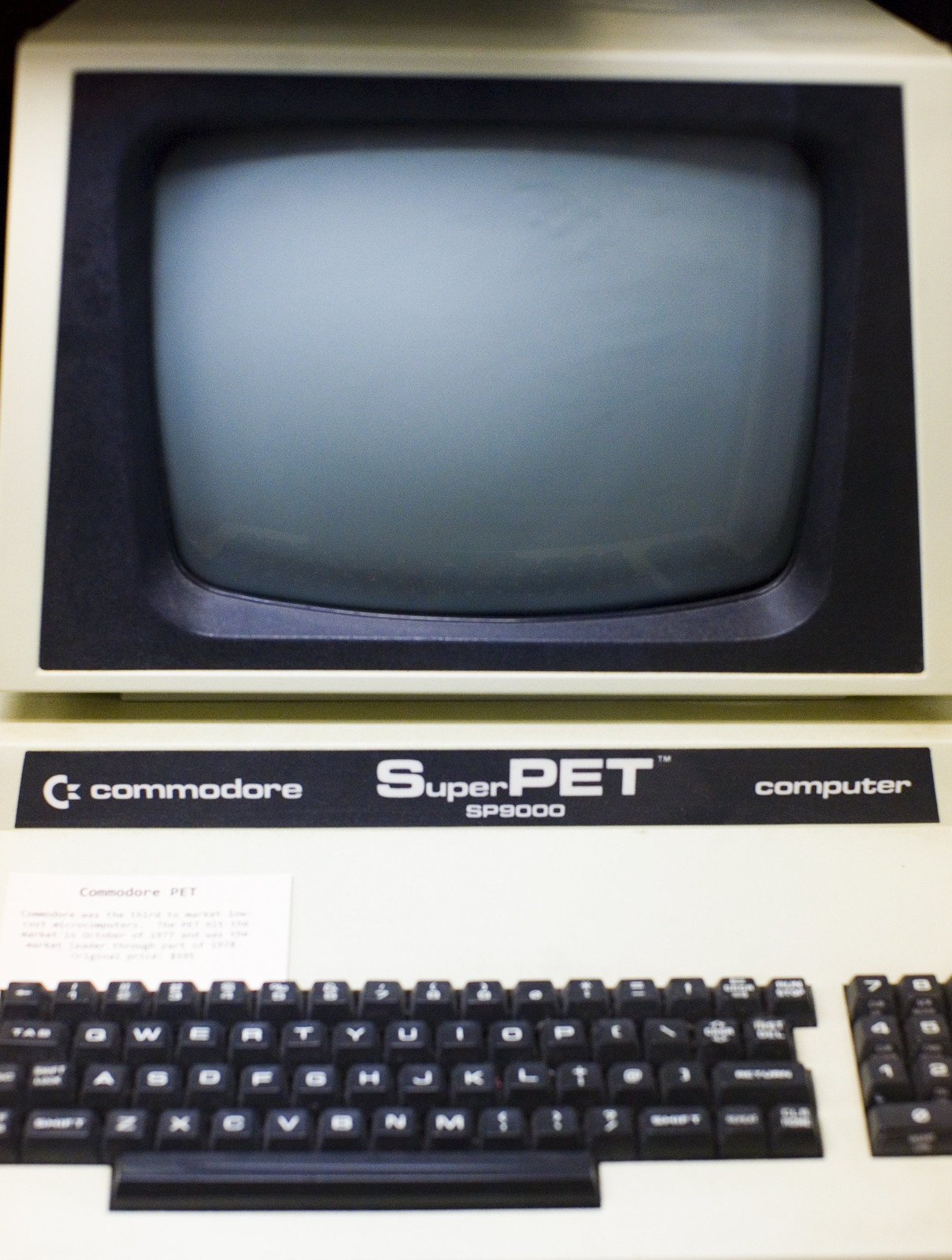This image showcases a vintage Commodore Super Pet SP9000 computer. Dominating the scene is the classic, large, old-fashioned screen, which is turned off, giving it a blue hue. The screen is encased in a white border, adding to the retro aesthetic. Directly beneath the screen is a black horizontal strip, prominently featuring the text "Super Pet SP9000" in the center, flanked by the Commodore logo on the left and the word "computer" on the right. Below this strip, a white paper partially blocks the view, only revealing the text "Commodore PET." The lower part of the image displays a black, QWERTY keyboard, though part of the number pad is cut off from the frame. The background of the picture is a simple white, emphasizing the computer's stark and historical design. Overall, it is a minimalist depiction of an iconic piece of computing history.